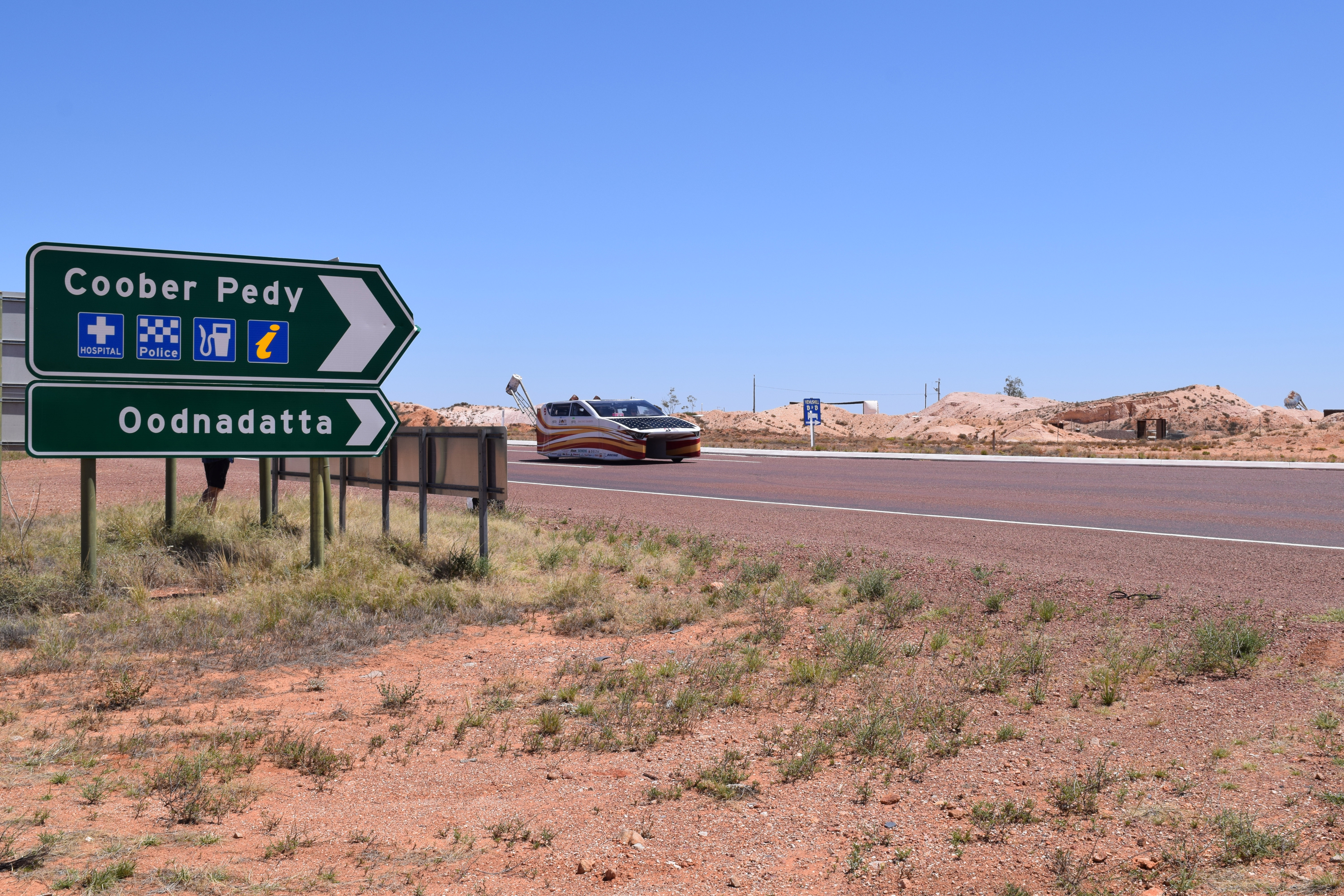In the arid desert landscape, likely somewhere in California or Arizona, a paved road stretches off into the distance beneath a bright blue sky. The dry terrain dominates the scene, punctuated by sparse, dying plants and rocky features. In the middle of the image, a road sign stands prominently. The sign reads "Coober Peedy" and "Oodnadatta," with directional arrows pointing right, indicating the way to a hospital, police station, gas station, and information center, all depicted with standard blue highway symbols. 

A white car with a futuristic design and unique features, including red, white, and yellow or orange stripes along its side and a peculiar tail-like structure at the back, possibly a parachute, travels from left to right on the asphalt road. This vehicle, resembling a cross between an SUV and a minivan but with an unconventional look, adds an intriguing element to the otherwise stark and dry desert scene.